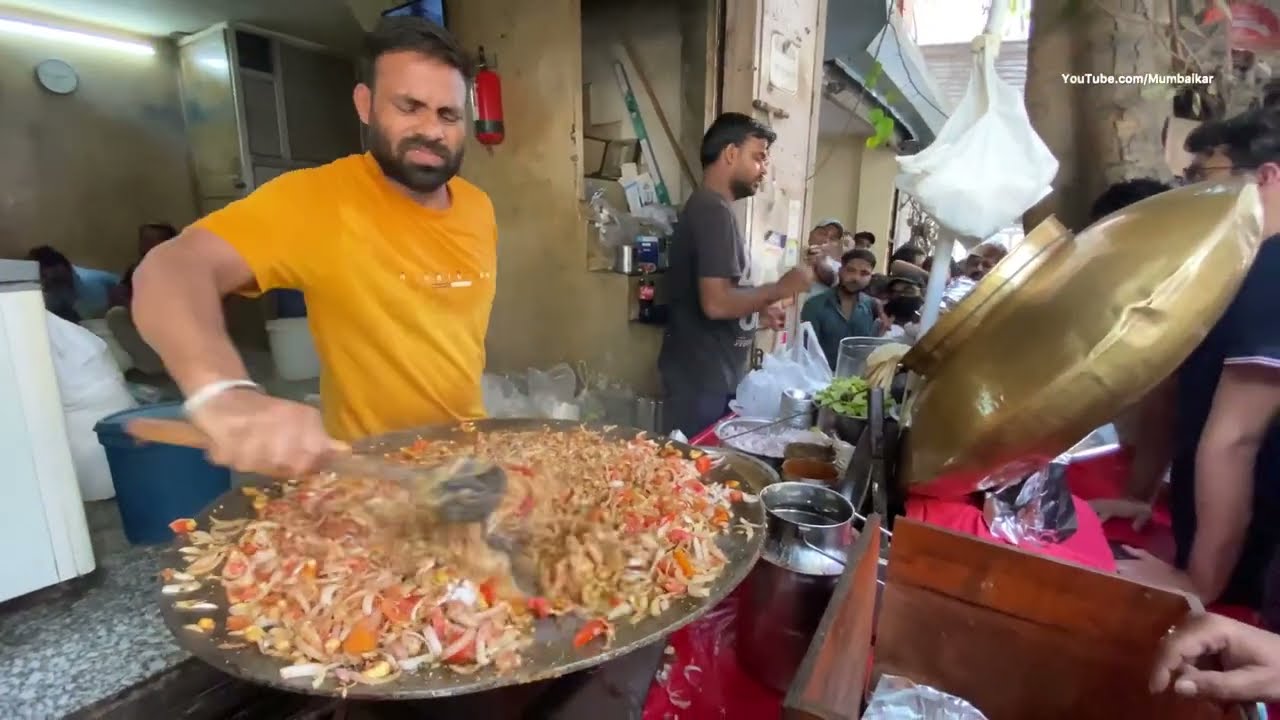In this vibrant scene, an outdoor street vendor chef is the central focus, engaged in rapid, skillful cooking on a large, round metal grill. The chef, a man of South Asian descent, is wearing a short-sleeved, goldenrod yellow t-shirt and a white bracelet on his wrist. His face, framed by a black beard and short black hair, is sweaty and intense as he stirs a medley of vegetables, including onions and colorful red and orange peppers, along with pieces of chicken. The motion of his large spoon or ladle is so fast that it appears blurry. 

Around him, there's a bustling atmosphere teeming with activity. To the right, another man dressed in a gray shirt, also with a black beard and hair, seems to be serving customers or handling carry-out orders, with plastic bags visible in front of him. Behind them, a crowded restaurant space can be partially seen, filled with people sitting and interacting, adding to the lively ambiance.

Other details flesh out the scene: a red fire extinguisher is mounted on the wall, a white clock is tucked away in the upper left corner, and a bottle of Coca-Cola is visible alongside fajita wrappers. The background is a hive of activity, with kitchen workers on break and perhaps a cashier handling transactions. The kitchen, though somewhat obscured, exudes a unique, bustling charm, reflecting the popularity and energy of the place.